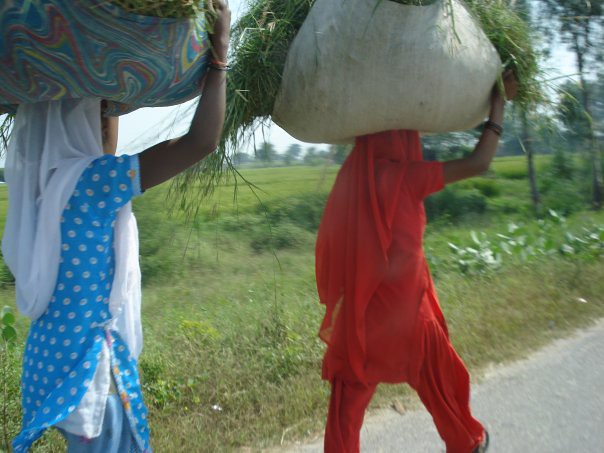This image depicts two women walking down a road adorned with lush vegetation, including trees, bushes, and wild grass on the left side. The women, who appear to be Indian, are each balancing large bundles of what seems to be grass or hay wrapped in cloth on their heads. The woman in the front is dressed in traditional Indian attire, consisting of a red salwar kameez with a matching dupatta draped over her head. She supports the large white sack with her right arm, which is adorned with a watch. Behind her, the second woman wears a blue and white salwar kameez with a white dupatta. She holds her similarly-sized sack, full of the same grass or hay-like material, with both hands. The women are photographed from behind as they walk down the road, their colorful attire standing out against the greenery.